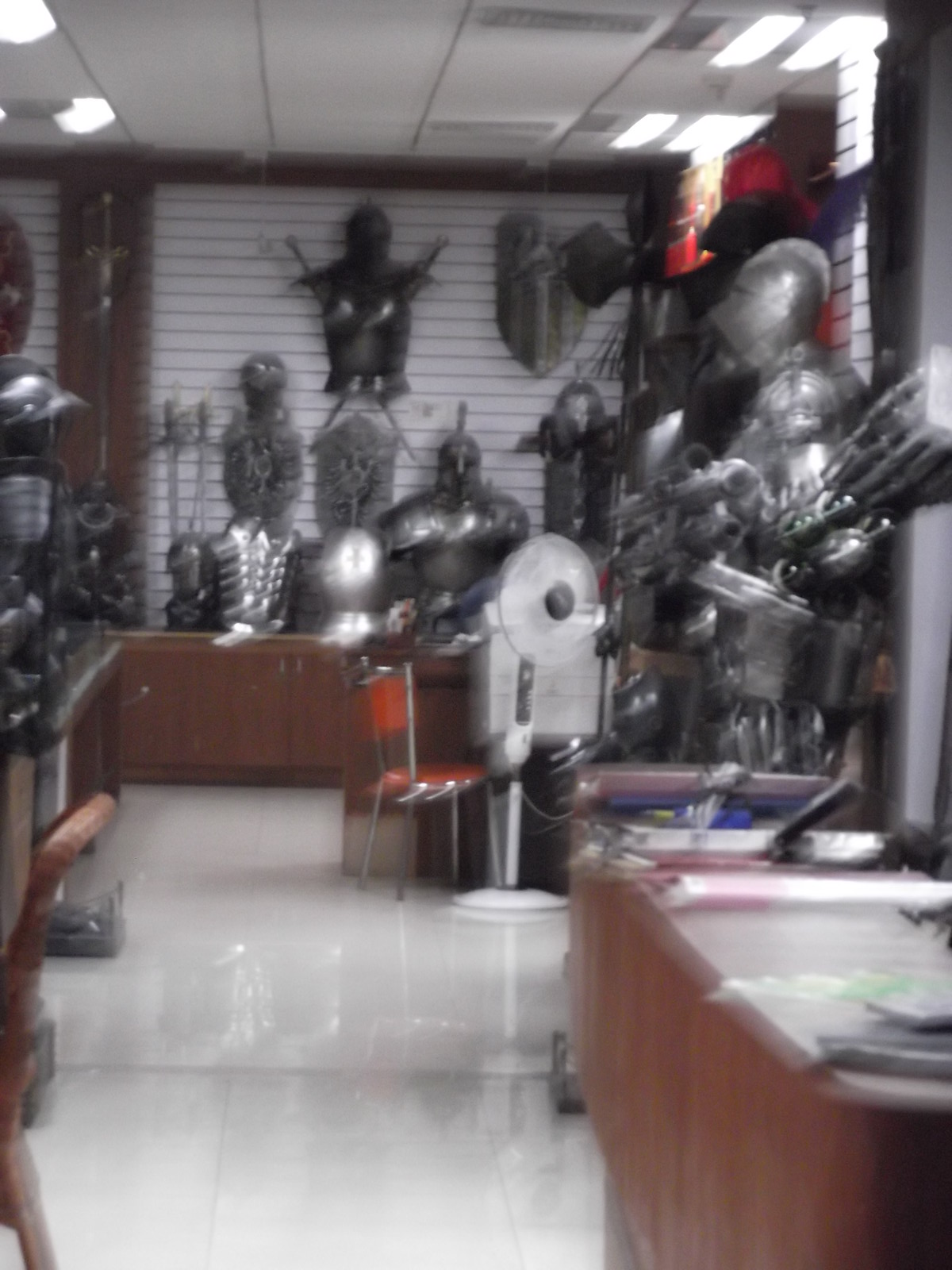This out-of-focus color photograph captures the interior of a shop displaying various medieval knight artifacts. Prominently on the left, there's a knight statue adorned in full armor. The back wall is decorated with a collection of metal masks, helmets, shields, and torso armor, reminiscent of the gear used by knights. Centrally positioned in the frame is a red chair with a metal base, alongside a white floor fan. The floor is a shiny white tile that reflects the store's bright fluorescent lighting. On the right, a brown counter or desk is positioned near a credit card kiosk. The right side also features a detailed display of a full set of knight's armor including a silver helmet and torso protection. Wooden paneling lines the display cases, and scattered throughout are various items enhancing the medieval motif of the store.